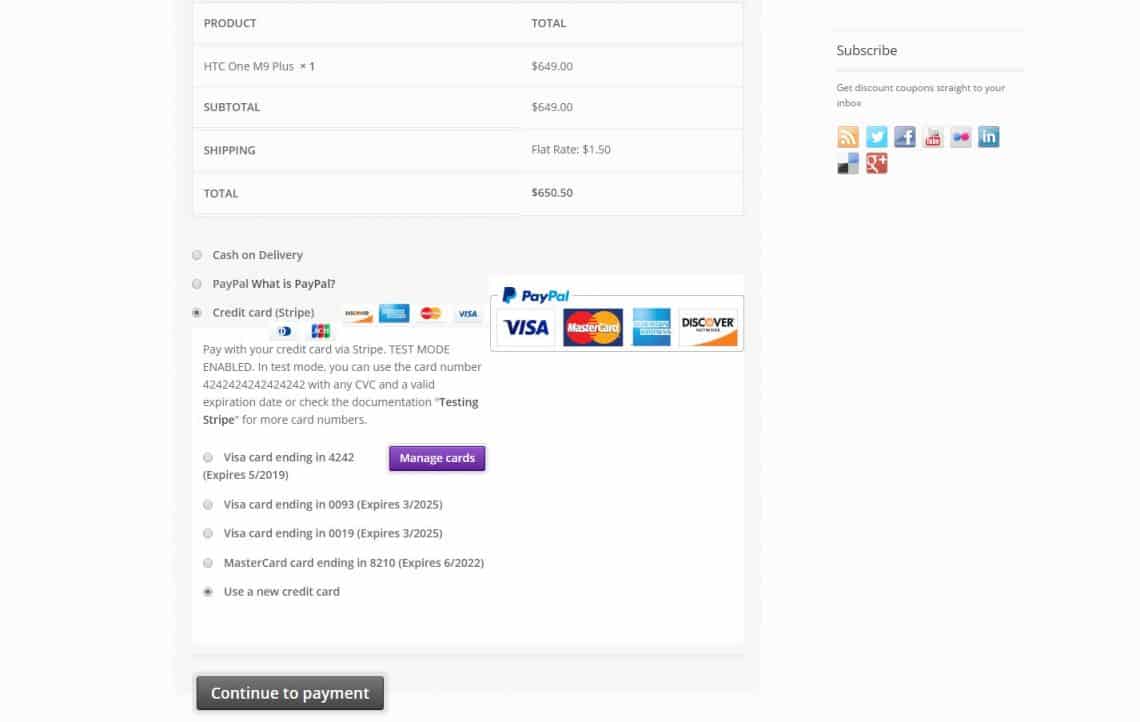This detailed image depicts the final page of an online product purchase, focusing on the summary and payment options. At the top, a header reads "Product Total." On the left side, there is a larger box displaying the product, while to the right is a smaller box labeled "Subscribe" with an invitation to receive discount coupons directly to your inbox. Below this are icons for various social media platforms, including Twitter, Facebook, Indeed, Google Plus, and others.

The main product listed is "HTC One M9 Plus," with a total price of $649. Below this, the breakdown states a subtotal of $649, a flat shipping rate of $150, leading to a total of $799.00. Several payment options are presented: "Cash on Delivery," "PayPal," with an accompanying explanation "What is PayPal," followed by "Credit Card"—specifically through Stripe (selected), indicating supported credit cards: Discover, American Express, MasterCard, and Visa, though these icons appear slightly blurry.

On the right side, larger images detail PayPal and various credit cards, reiterating support for Visa, MasterCard, American Express, and Discover. Additional information about paying with a credit card leads to a pulled-up Visa card option for completing the purchase.